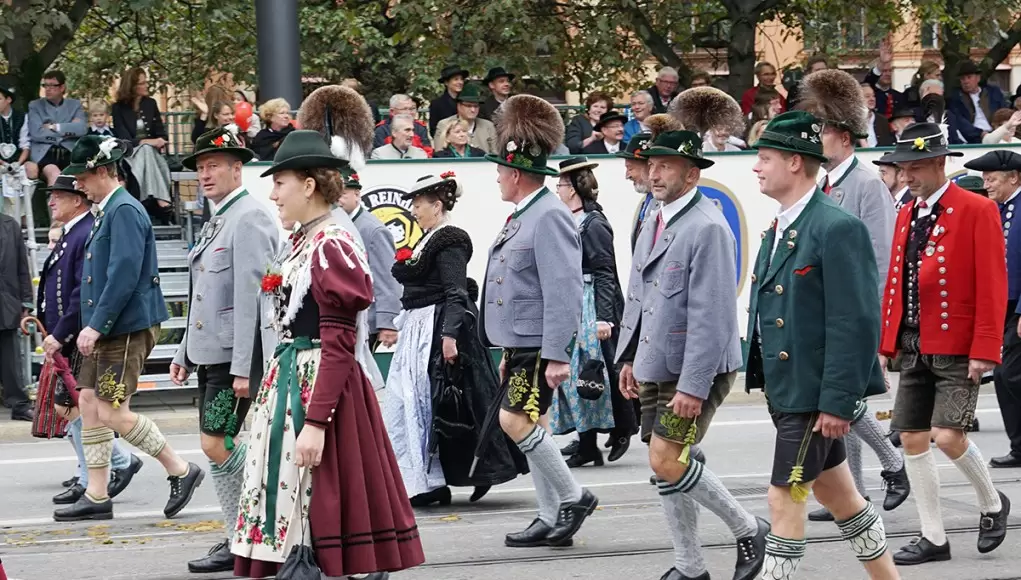This landscape-style photograph captures a vibrant parade, possibly part of a cultural heritage festival, where participants are dressed in traditional German attire. Men and women of various ages walk a road lined with trees, parading in front of spectators seated on bleachers. The men don colorful jackets in red, navy, hunter green, and gray, paired with knee-length shorts, special knitted stockings, and fancy dress shoes. Each man also wears a small green hat adorned with feathers or flowers. The women wear full-body dresses adorned with aprons and shawls tied around their shoulders, fastened with a red rose or similar flower. Their outfits include maroon, purple, black, and green dresses, some featuring collars and intricate designs. The women's headwear varies, with some sporting green caps with feathers and others wearing white hats. A partially visible sign and a large banner with indistinct logos add to the festive backdrop of the parade.